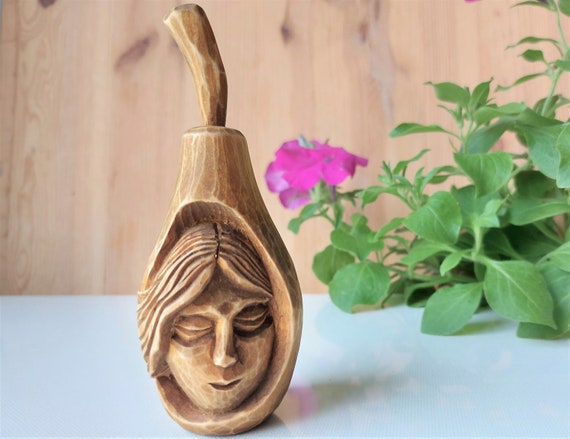This photograph features a detailed wooden sculpture of a pear with a girl's face intricately carved into the front. The girl's face has closed eyes and long hair that is parted down the middle, flowing gracefully around the pear-shaped figure. The sculpture, which has a small stem, sits on a pristine white table or counter. The backdrop consists of unpainted wood paneling or shiplap, adding a rustic feel to the scene. To the right of the sculpture, a pink petunia with lush green leaves adds a touch of color to the earthy tones of the image.